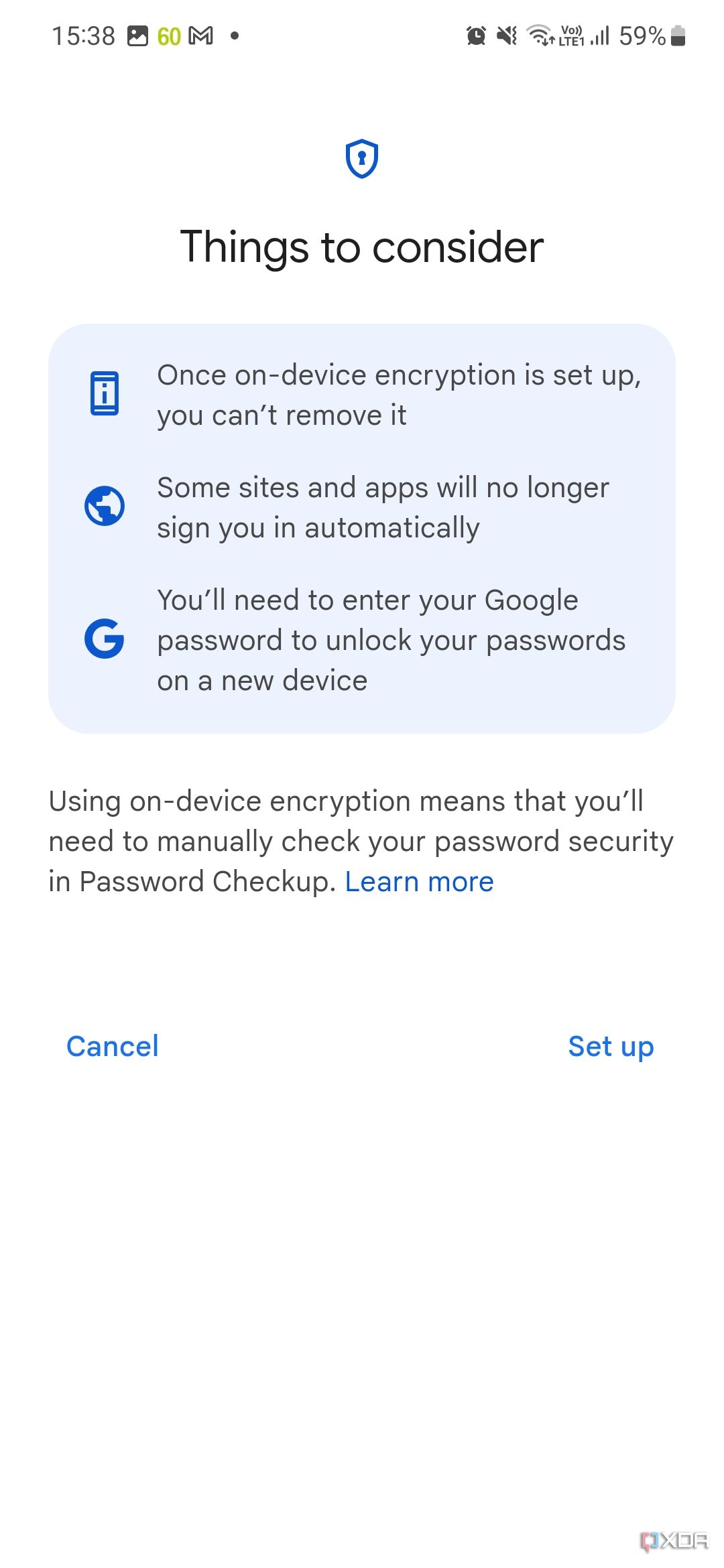This screenshot was taken from a cell phone at 3:38 PM, as indicated in the upper left corner. The battery is at 59% and multiple notifications are visible in the top toolbar. 

The screenshot captures a webpage with a predominately white background and a blue key lock symbol centered in the upper section. Below the symbol, the text reads "Things to Consider," followed by a gray highlighted square containing the message: "Once on-device encryption is set up, you can't remove it. Some sites and apps will no longer sign you in automatically. You'll need to enter your Google password to unlock your passwords on a new device."

Further down, the webpage states, "Using on-device encryption means that you'll need to manually check your password security and password checkup," followed by a "Learn more" link.

At the very bottom of the screenshot are two buttons: "Cancel" on the left and "Setup" on the right, indicating that this is the initial step for setting up encryption on the phone.